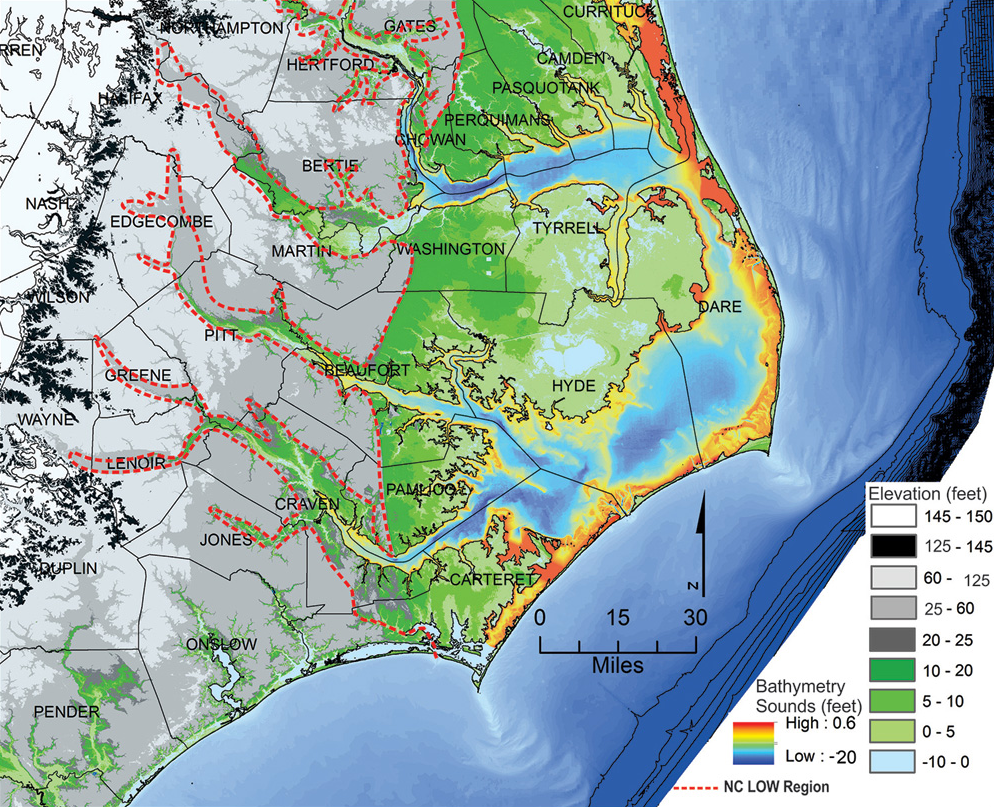This image is a detailed geographical map showcasing the coast of North Carolina, specifically highlighting Pamlico Sound. The map is divided into counties, such as Hyde, Dare, Camden, Tyrell, Martin, Bertie, Edgecombe, Craven, Jones, Onslow, Carteret, Greene, Hertford, Gates, and Northampton. The map is color-coded to indicate various elevations and depths, with a legend in the lower right-hand corner showing measurements in feet. The left side of the map includes elevations that rise into a mountainous region, while the right side, marked by a dotted line, displays bathymetric measurements, illustrating the ocean's depth along the coastline. This dotted line underscores the division between North Carolina's low-lying regions and the higher elevations.